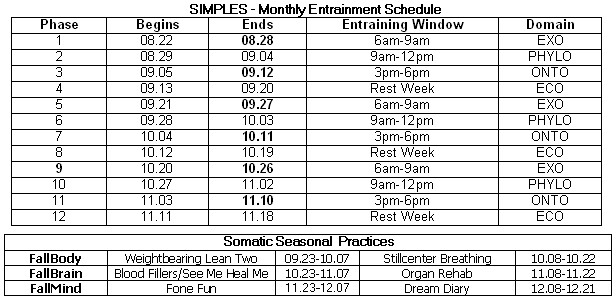The image depicts a black and white printed schedule titled "SIMPLE'S Monthly Entrainment Schedule," laid out on a white background in small uppercase print. The table is divided into 12 rows, each labeled sequentially from Phase 1 to Phase 12. Each row includes detailed columns labeled "Phase," "Begins," "Ends," "Entraining Window," and "Domain." The "Begins" and "Ends" columns specify the start and end times for each phase, typically ranging from 10 to 30 minutes. The "Entraining Window" lists broader time ranges such as 6 to 9 a.m. and 9 to 12 p.m., while the "Domain" column alternates among categories such as "Exo," "Phylo," "Onto," and "Eco."

Beneath this primary table, there's another section titled "Somatic Seasonal Practices," which is organized into three rows: "Fall Body," "Fall Brain," and "Fall Mind." Each row appears to list various dates and activities, such as "Organ Rehab" and "Dream Diary," likely indicating a series of courses or sessions with specified times. The meticulous layout and detailed information resemble a structured Excel sheet, emphasizing both scheduling and thematic entrainment practices.